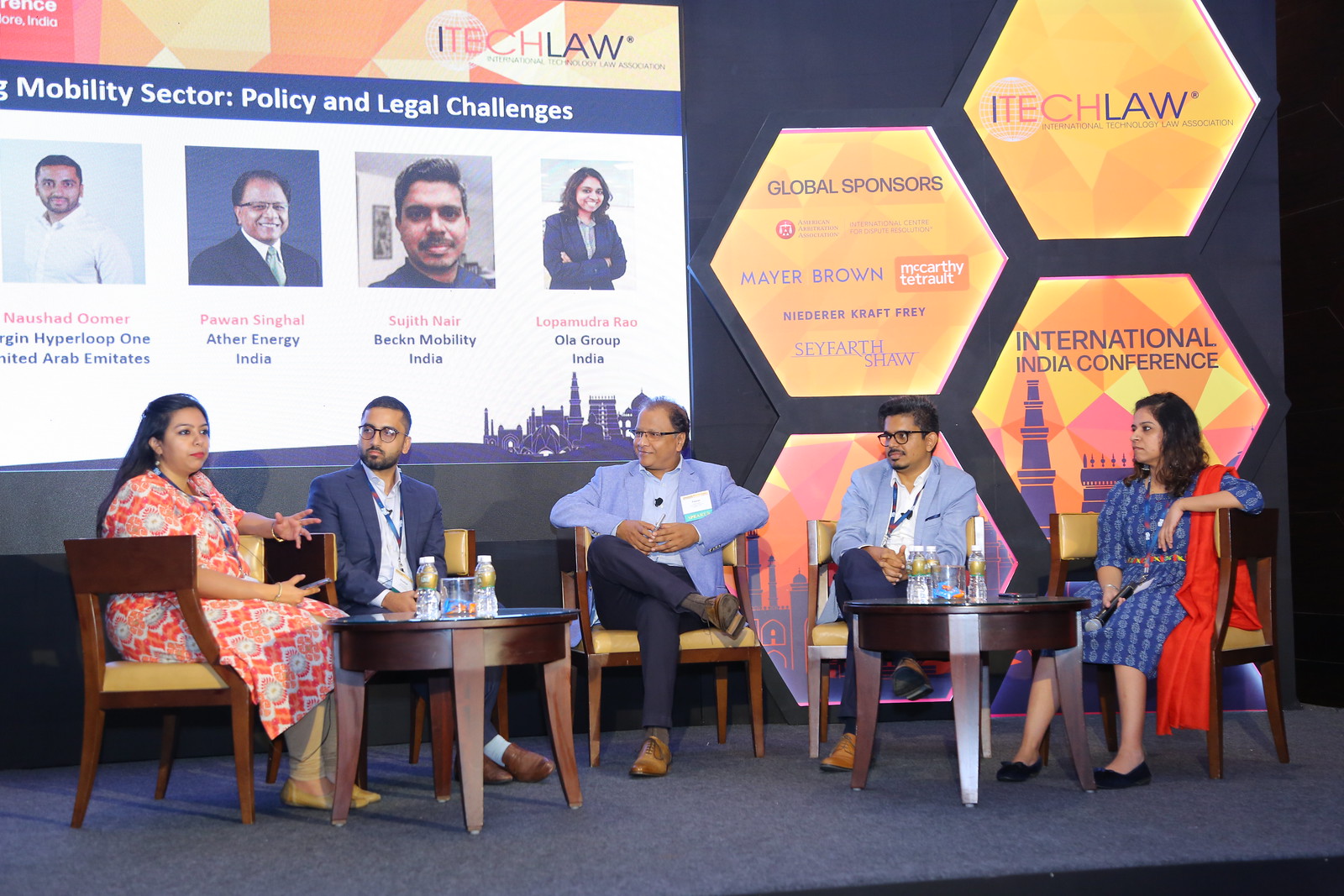At an International India Conference presented by iTechLaw, five panelists are seated on a stage against a backdrop displaying participant photographs and names, including Nashad Omar, Pawan Singhai, Sijuth Nair, and Lopamudra Rao. They are supported by global sponsors Mayer Brown, Niederberger Kraft Frey, Seyfarth Shah, and McCarthy Tetreault. 

From left to right, the panelists are as follows: 

1. A woman in a vibrant orange, white, and blue dress with long black hair, hands raised slightly—one hand holding a phone in her lap—sits on a wooden chair with a yellow seat.
2. A man with short black hair, brown skin, black glasses, and a blue jacket over a light blue shirt, wearing a lanyard, looks at the woman to his left while seated behind a circular table.
3. The middle panelist, wearing a light blue jacket and matching shirt with blue jeans, has his legs crossed and sits with no table in front of him.
4. Another man with dark black hair, brown skin, black glasses, a black mustache, and goatee, clad in a light blue jacket and white shirt, gestures towards the left, with a circular table in front of him.
5. Lastly, a woman in a blue dress with curly black hair cascading beside her face, partially covering her ears, holds a microphone in her lap and rests another hand on the chair’s armrest.

The background features a banner titled "Mobility Sector Policy and Legal Challenges" and several hexagons indicating "Global Sponsors," "IETCE Law," and "International India Conference."